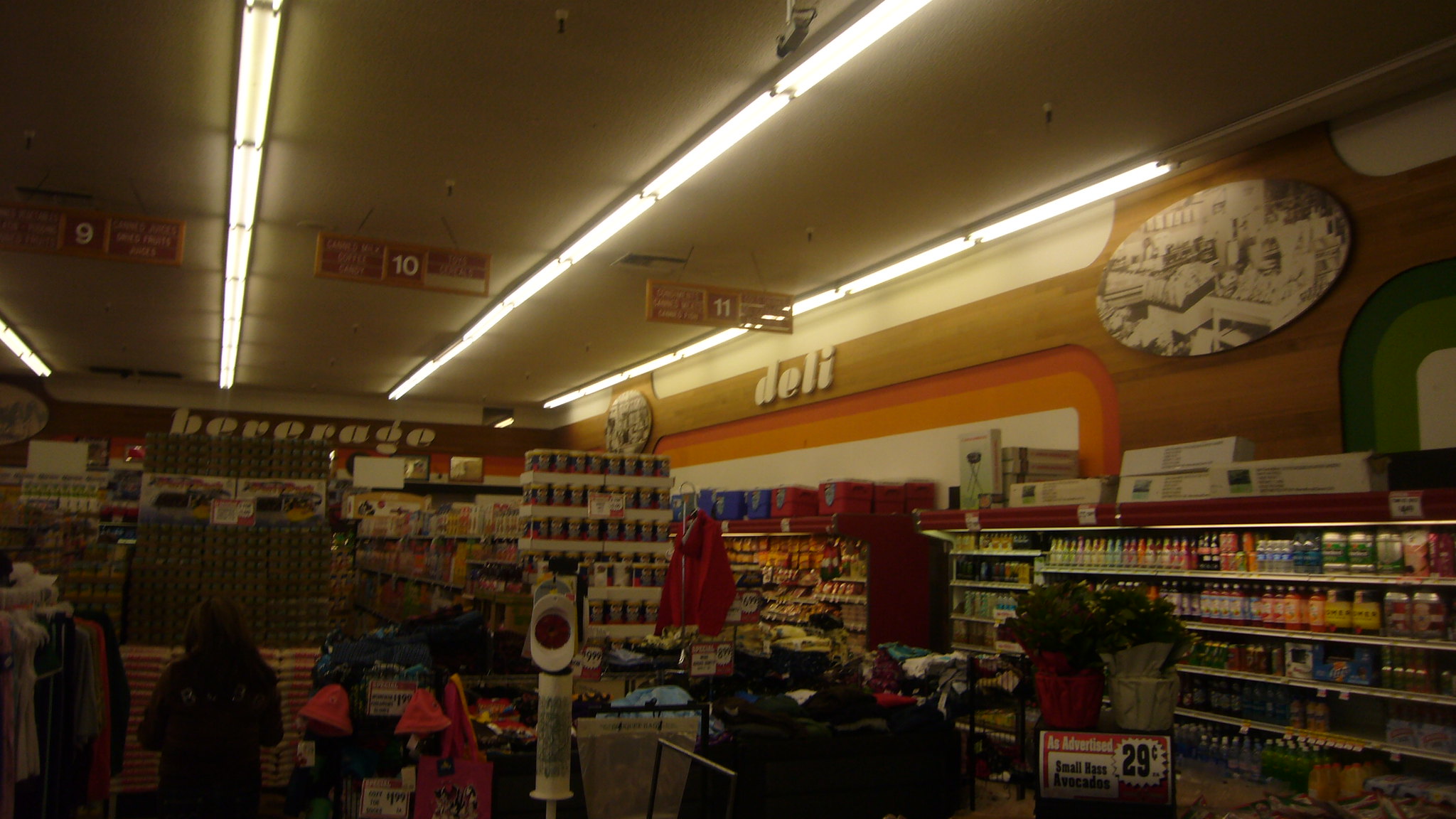The image portrays the interior of a retail store, encapsulated within a rectangular frame. The ceiling, which is painted white, features four linear light strips illuminating the scene with a bright, white glow. Suspended from the ceiling, there are three red signs with bold, white numerals indicating aisle numbers: 9 on the far left, 10 in the center, and 11 on the right. In the background, the word "Beverage" is prominently displayed, suggesting the section of the store designated for drinks.